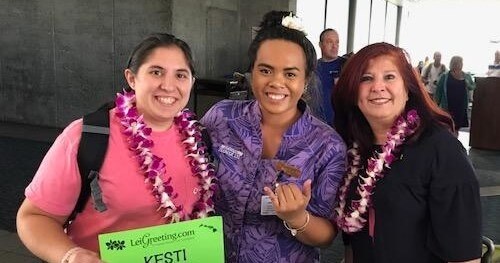This is a horizontally oriented, realistic photograph capturing three women in the foreground with a background that suggests an airport or hotel, filled with a few people walking around. The focus of the image is on the three women, all smiling and adorned with traditional Hawaiian leis made of dark pink and purple flowers.

On the left, there is a young woman in her 20s with light brown skin and black hair, who appears to be Hispanic. She is smiling warmly and wearing a pink shirt along with a backpack. She holds a neon green sign that reads "Leyi Greetings Kesti."

In the middle stands an African American woman, possibly in her late 20s or early 30s. She is dressed in a purple shirt adorned with a badge featuring white text. A flower decoratively rests in her hair, and she is making a cheerful hand gesture.

On the right is a white woman, likely in her 30s or 40s, with striking red hair. She is also smiling and wearing a black cardigan. Both her and the woman on the left have matching leis.

The background, while not the main focus, includes a glimpse of a stone or concrete wall on the left and several travelers on the right, including a man in a blue shirt and a woman in a black shirt with a green jacket. Their casual presence adds context, hinting that the photograph might have been taken as the women arrived at their destination, possibly receiving their leis as a welcome gesture.